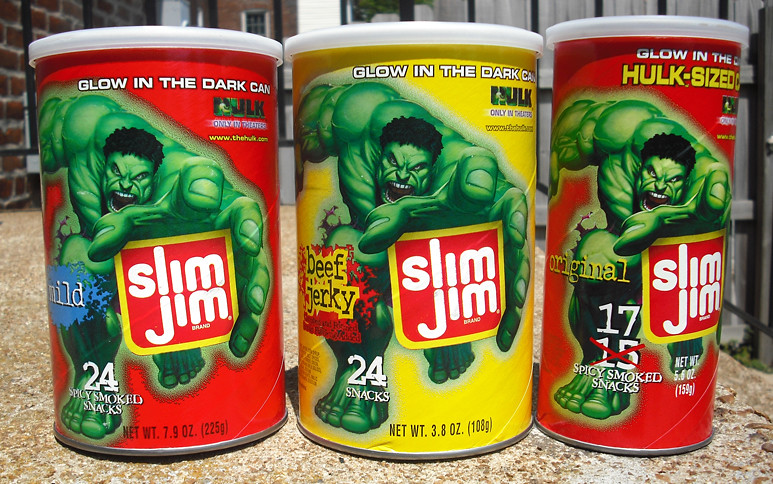This is a photograph of three Slim Jim containers neatly arranged on a brown and white marbled granite countertop. Each container features a prominent image of the green, angry Hulk, who appears to be reaching out towards the Slim Jim logo. The containers are tall and slim with white lids, and the top of each can displays the text "glow in the dark can" written in white. 

Starting from the left, the first container has a red background with the word "mild" on it. It holds 24 snacks, indicated by white text on the bottom left corner. The middle container has a yellow background and is labeled "beef jerky" in black font. This container also holds 24 snacks. The container on the right is slightly thinner and taller than the others, with a red background and labeled "original." Initially marked for 15 snacks, this number is crossed out with a red X and corrected to 17 snacks.

The green Hulk character dynamically reaches towards the Slim Jim logo on each container, tying the visually striking design elements together against the varied, vibrant backgrounds.